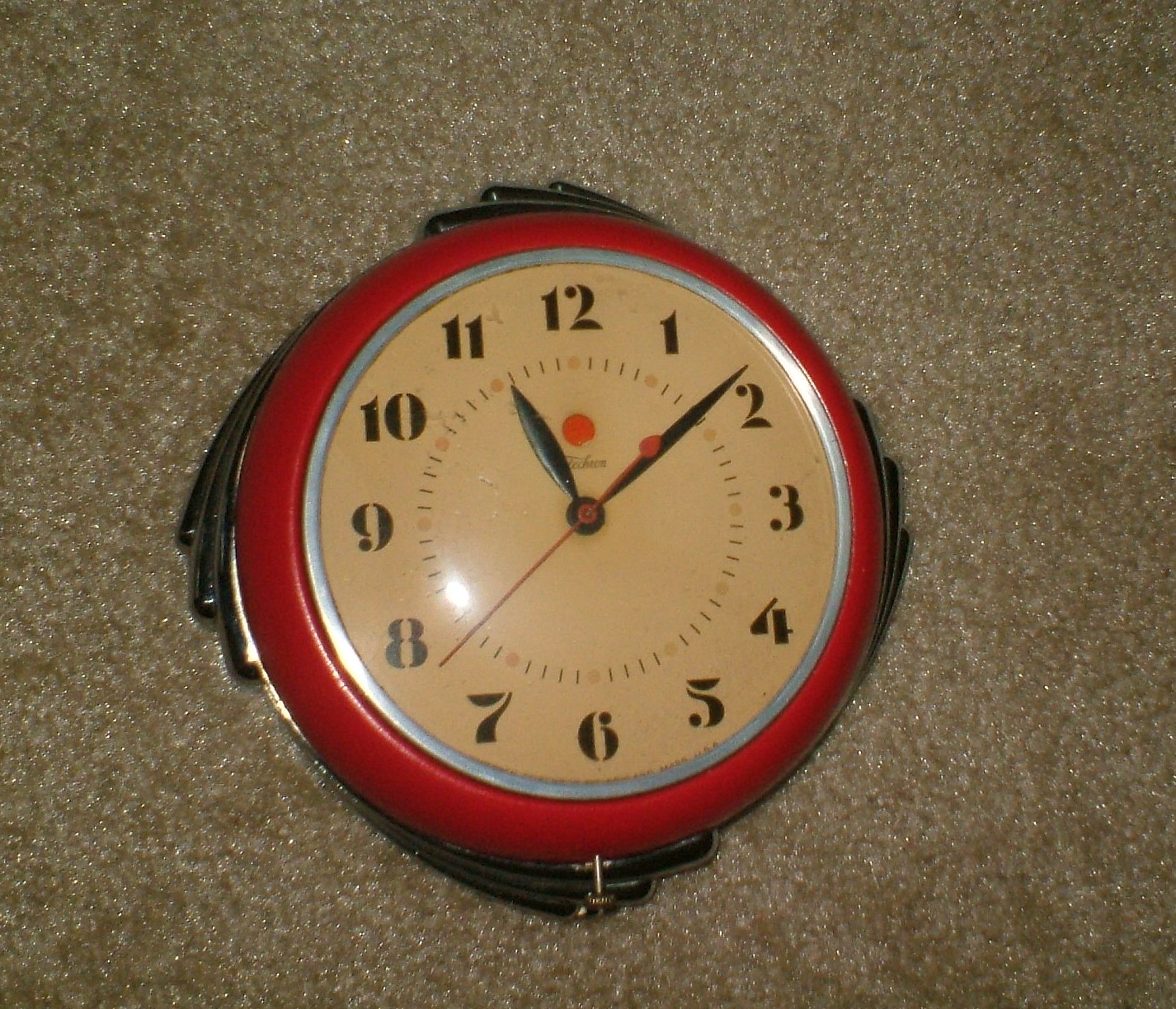The image features an old-fashioned circular clock lying on a soft, beige, textured carpet. The clock has a red border and an intricate design at each cardinal direction, consisting of three concentric silver waves. It has an orangey interior face rimmed in silver within the red border. The numbers 1 through 12 are positioned around the circumference of the clock's face. There are two main hands and a slim, red second hand. The time shown on the clock is approximately 11:08, with the second hand pointing to around 38 seconds.